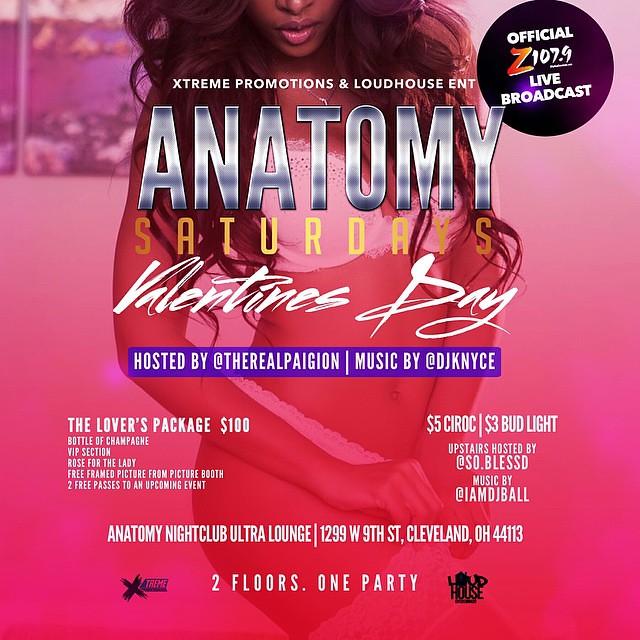This is a detailed, full-color digital advertisement primarily featuring shades of pink. It promotes a Valentine's Day event at the Anatomy Nightclub Ultra Lounge in Cleveland, Ohio. The focal point of the poster is the semi-profile image of a darker-skinned woman with long, voluminous curly brown hair, pink lipstick, and very full lips; her image fades under a pink shade. She is dressed in a white bra, with her hands positioned in front of her. 

The advertisement prominently announces an official Z107.9 live broadcast and includes various promotions organized by Extreme Promotions and Loud House Entertainment. The event, titled "Anatomy Saturdays," offers a special lover's package for $100, which includes champagne, VIP access, and roses. In addition, the advertisement mentions entertainment details, with a purple bar highlighting that the event is hosted by @TheRealPage and features music by @DJKNyce. Additional critical information is presented in white letters within a dark purple and black circle, ensuring clarity and emphasis.